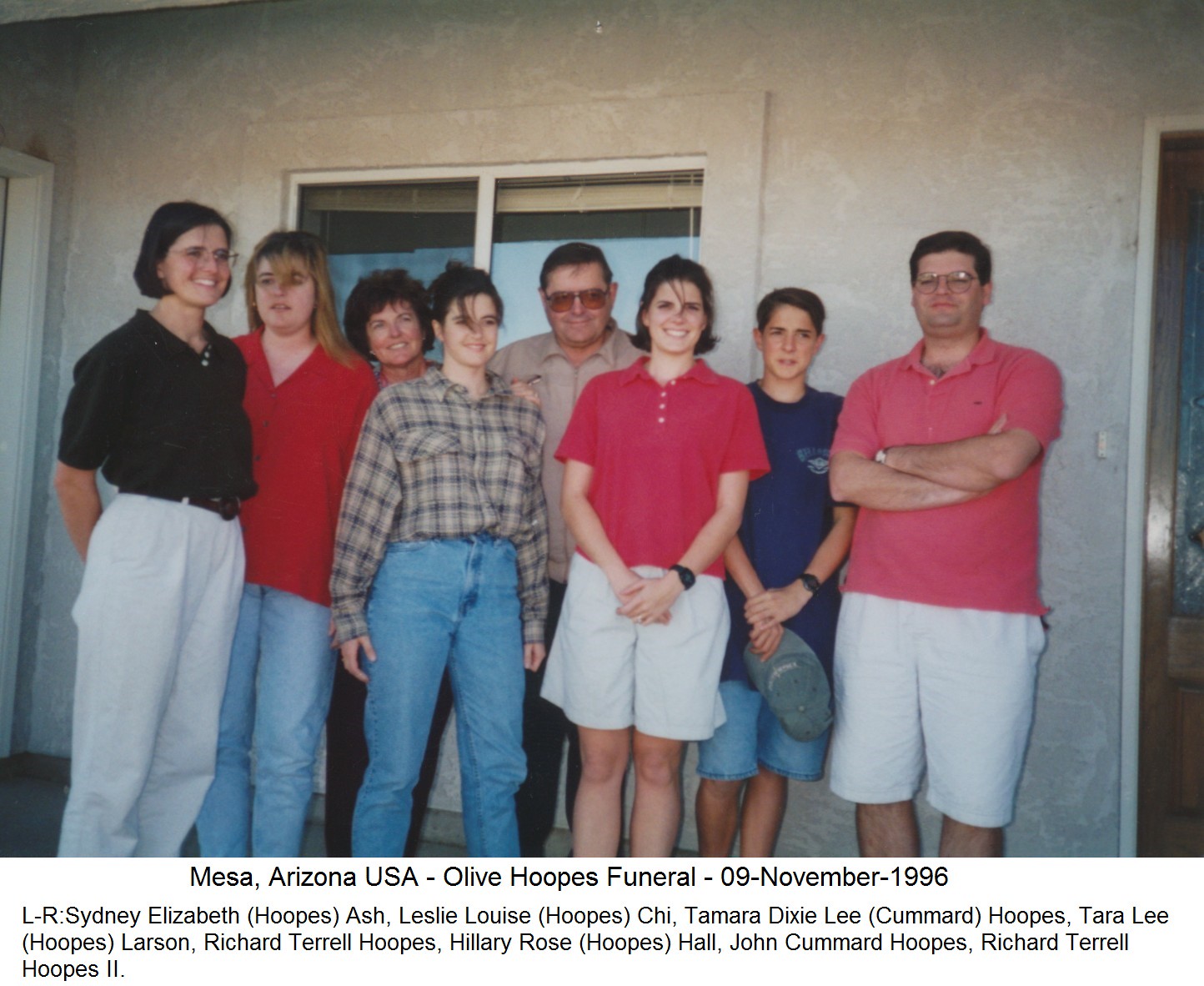The image is an outdoor photograph taken during the daytime in front of a gray stone building, likely during a funeral service. The caption reads: "Mesa, Arizona, USA - Olive Hoops Funeral - 09 November 1996." It features eight family members named from left to right: Sidney Elizabeth (Hoops) Ash, Leslie Louise (Hoops) Chi, Tamara Dixie Lee (Cummerd) Hoops, Tara Lee (Hoops) Larson, Richard Terrell Hoops, Hillary Rose (Hoops) Hall, John Cummerd Hoops, and Richard Terrell Hoops II.

From left to right, the individuals are positioned as follows:
1. Sidney Elizabeth, a young woman with short brown hair wearing a black shirt and white pants, is smiling and looking to her right.
2. Leslie Louise, with long blonde hair, wearing a red shirt and blue jeans, is facing the camera.
3. Tamara Dixie Lee, an older lady with short curled hair, slightly hidden but smiling.
4. Tara Lee, in a plaid shirt and blue jeans, stands in a spread-leg stance with arms by her sides.
5. Richard Terrell, an older man with short brown hair and tinted glasses, slightly larger in size and smiling directly at the camera.
6. Hillary Rose, a young woman in her 20s with a red shirt and white pants, smiling directly at the camera.
7. John Cummerd, a teenage boy wearing a blue shirt and denim shorts, holding a baseball cap, looking slightly to his right.
8. Richard Terrell II, a man with clear glasses, a collar pink shirt, and white shorts, with arms crossed and eyes closed.

The family members appear composed and are mostly smiling, standing together outside, possibly in front of a church. This snapshot from 1996 captures a moment of shared togetherness during a solemn event.